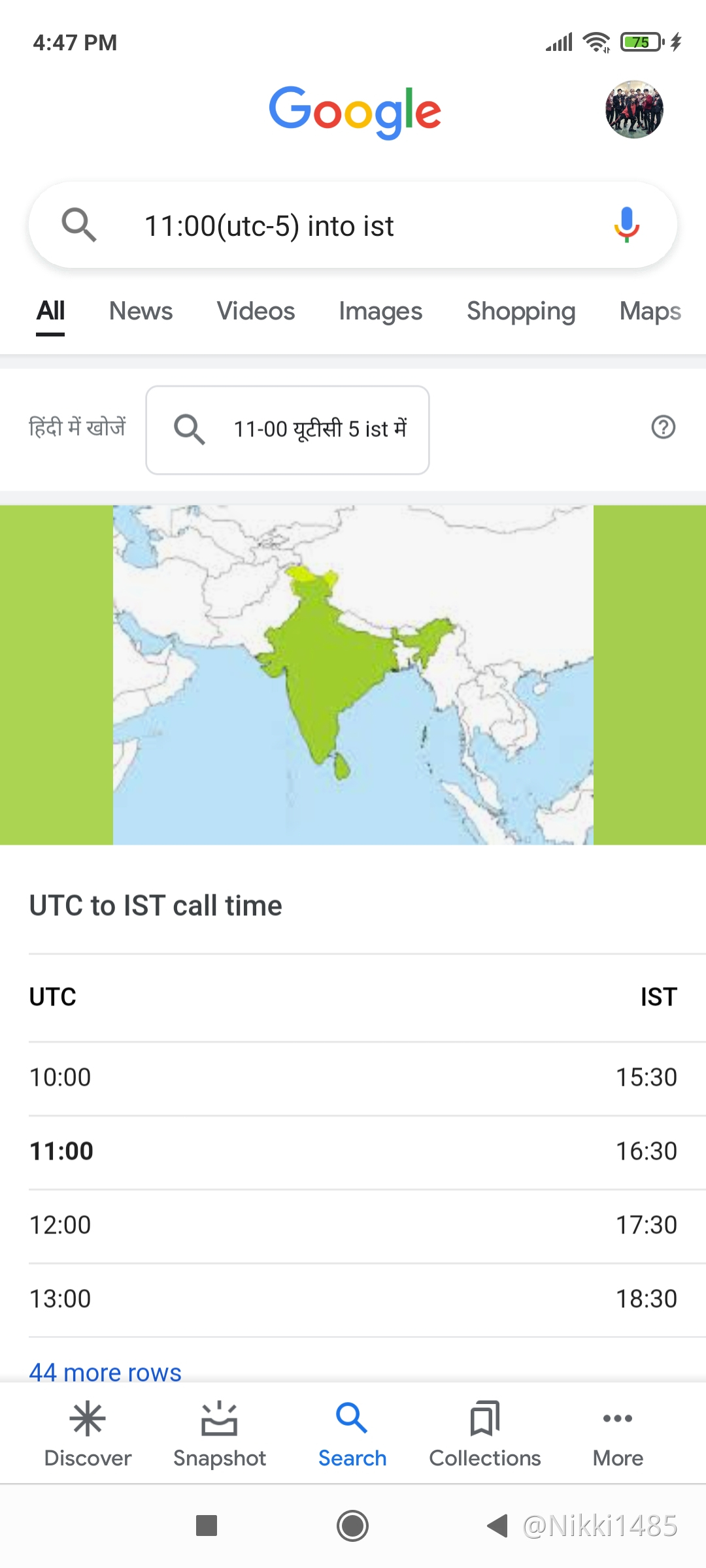This image captures a screenshot of a mobile Google web search page. At the top left corner, the phone displays the current time. Adjacent to this on the right, icons indicate the device’s signal strength, Wi-Fi strength, battery percentage, and a lightning bolt showing the phone is charging. Centered at the top is the Google logo on a white background, with the user's profile photo in a circle on the far right.

Below the logo, the search bar contains the query "11 o'clock utc minus five into ist." Directly beneath the search bar is a horizontal row of categories including "All," "News," "Videos," "Images," "Shopping," and "Maps," with the "All" category highlighted. 

Following this, the search results display a map and a list of times converting UTC to IST, arranged vertically: 
- 10:00 - 15:30
- 11:00 - 16:30
- 12:00 - 17:30
- 13:00 - 18:30